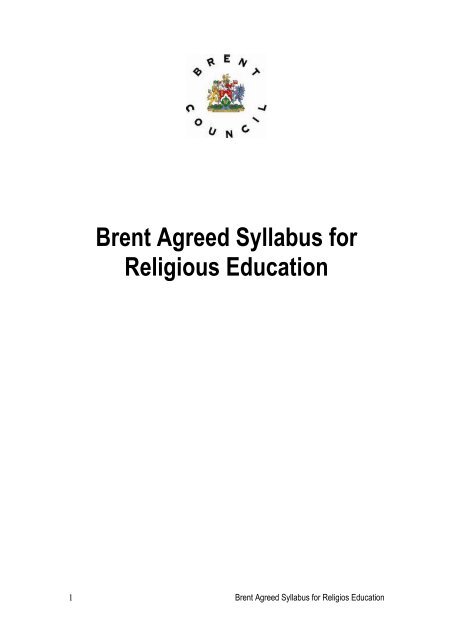The image depicts a predominantly white page, likely the first page of a student handbook or school document. At the top of the page, "Brent Council" is written in small text, with a colorful crest or logo beneath it featuring red, green, purple, yellow, and blue elements. The exact design of the logo is unclear from the image but appears to resemble a bush, tree, or possibly a building with trees in an artistic style. Centrally positioned is the main text, "Brent Agreed Syllabus for Religious Education," in a larger black font, making it the focal point. At the bottom of the page, the same phrase, "Brent Agreed Syllabus for Religious Education," appears again in small text. Additionally, there is a small black line or the number "1" situated in the bottom left corner. The overall layout suggests a formal and minimalist design, emphasizing the title of the document.